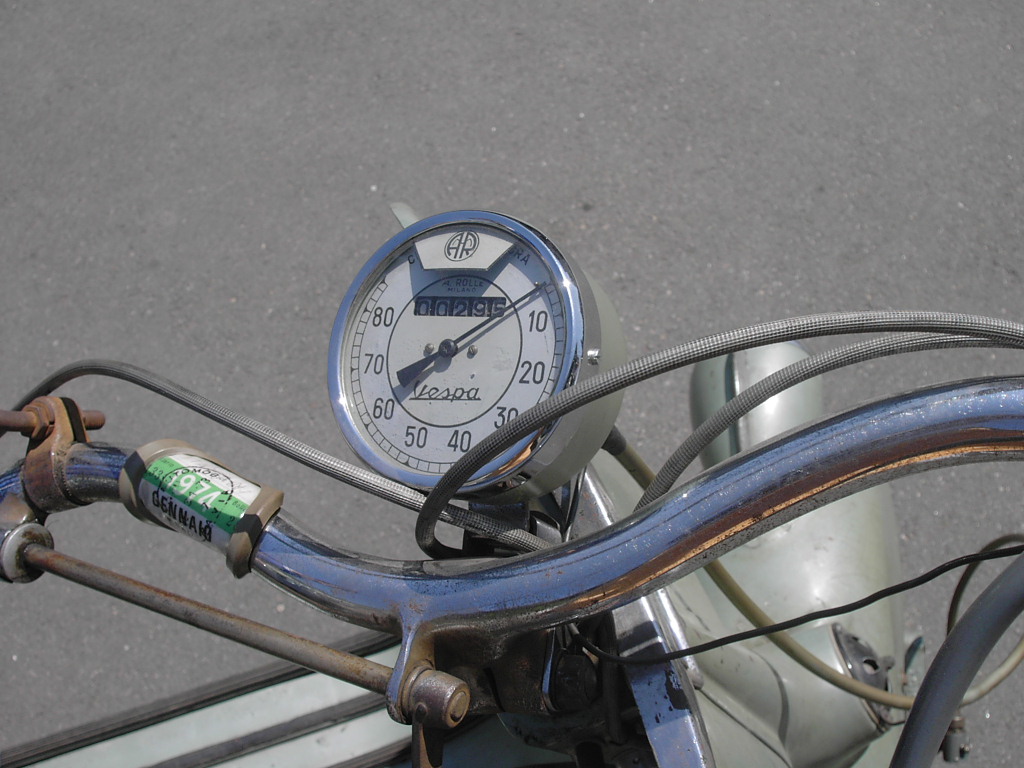The image captures a detailed, downward view from the perspective of someone seated atop a Vespa scooter. The clear, blue-tinted handlebars prominently frame the scene, with a circular odometer stationed right above them. The odometer, which features a blue outer rim, displays a mileage reading of 00295. Within the odometer, a speedometer marked in increments of 10, ranging from 10 to 80, features a needle currently pointing to zero, indicating the Vespa is stationary.

The background displays a black and grayish expanse of pavement, accentuating the foreground details. On the left handlebar, a small green sticker or emblem bears the text "1974 Geneva," with "Geneva" inscribed in black and possibly "G6MMA" following it. Additionally, a gray rod is visible, attached to the left-hand side, hinting at more intricate engineering details.